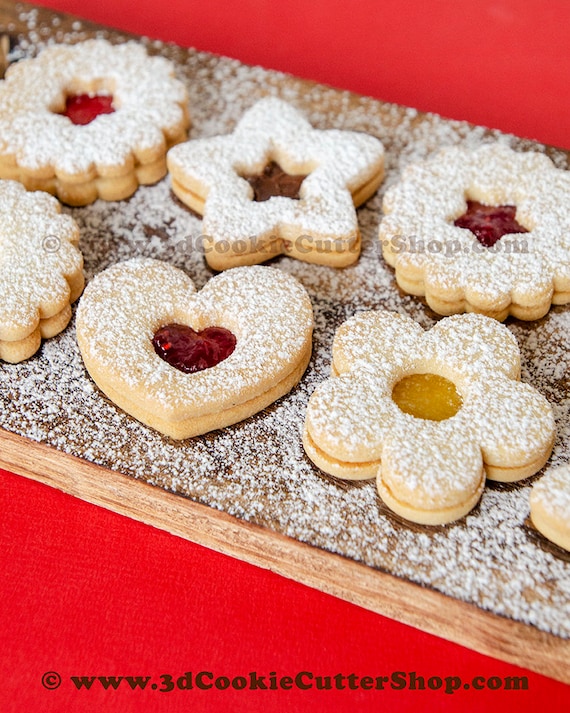This advertisement features a tantalizing array of cookies showcased on a wooden board, promoting the website www.3dcookiecuttershop.com. The image displays six intricately shaped sugar cookies, including hearts, flowers, and stars, each adorned with powdered sugar. These cookies are sandwich-style, with vibrant jam fillings peeking through their center indentations—the heart has a red heart-shaped jam insert, the flower has an apricot-colored circular filling, and the star displays a brownish filling. Set against a red background, this scene evokes a festive, holiday atmosphere, highlighting the delightful, handmade quality of the cookies, making them look delicious and inviting.